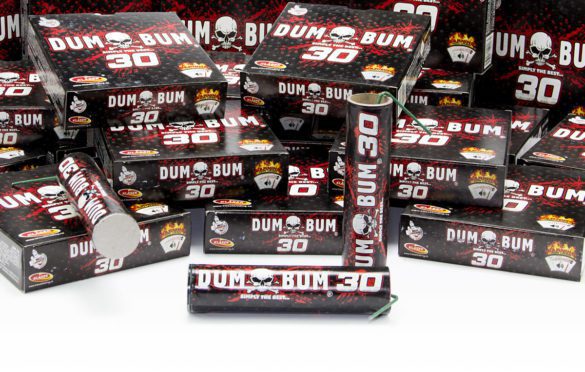The image displays a series of boxes labeled "Dumb Bum 30," prominently featuring a skull and crossbones between the words "Dumb" and "Bum." Each box, with its black background, white text, and red highlights, is laid out on a white counter, arranged in a horseshoe shape around the camera's viewpoint. Some boxes are open, revealing their contents: cylindrical firecrackers that resemble rolls of coins. These firecrackers replicate the box design with black backgrounds, white fonts, and red accents, and each has a green fuse extending from one end. The number 30 on the boxes suggests they may contain 30 individual firecrackers.